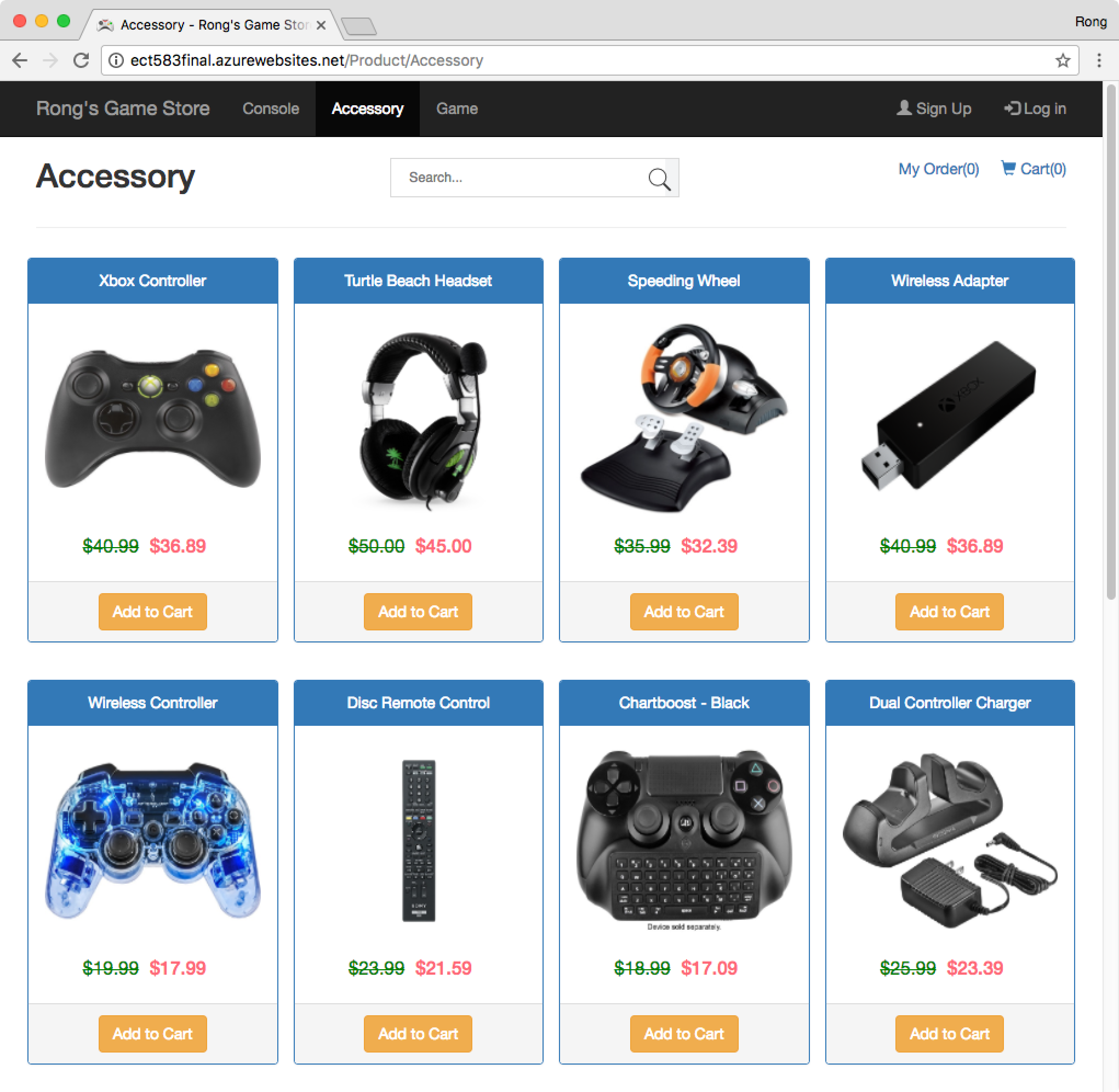This is a detailed description of a screenshot from the Accessory-Wrongs Game Store webpage, accessible at the URL ect58final.azurewebsites.net/product/accessory. At the top of the webpage, there is a black navigation bar with categories labeled "Wrongs Game Store," "Console," "Accessory," and "Game," with the "Accessory" tab highlighted. Directly below, the heading "Accessory" is prominently displayed in black text.

The page is divided into two rows, each showing four different gaming-related accessories with their corresponding images, descriptions, prices, and "Add to Cart" buttons.

**First Row of Accessories:**
1. **Xbox Controller:** 
   - Image: Xbox controller
   - Price: $36.89
   - Purchase Option: "Add to Cart" button

2. **Turtle Beach Headset:**
   - Image: Black headset
   - Price: $45.00 (in red text)
   - Purchase Option: "Add to Cart" button

3. **Speeding Wheel:**
   - Image: Steering wheel with two gas pedals on a black base
   - Price: $32.39
   - Purchase Option: "Add to Cart" button

4. **Wireless Adapter:**
   - Image: Wireless adapter
   - Price: $36.89 (in red text)
   - Purchase Option: "Add to Cart" button

**Second Row of Accessories:**
1. **Wireless Controller:**
   - Image: Controller with blue and clear exterior
   - Price: $17.99
   - Purchase Option: "Add to Cart" button

2. **Disc Remote Control:**
   - Image: Black remote
   - Price: $29.59
   - Purchase Option: "Add to Cart" button

3. **Chart Boost Black:**
   - Image: Apparent remote control
   - Price: $1709.00
   - Purchase Option: "Add to Cart" button

4. **Dual Controller Charger:**
   - Image: Dual control charger
   - Price: $23.39 (in red text)
   - Purchase Option: "Add to Cart" button

Each item is displayed with a clear image and concise labeling, with prices prominently shown and easily accessible "Add to Cart" buttons for convenient shopping.